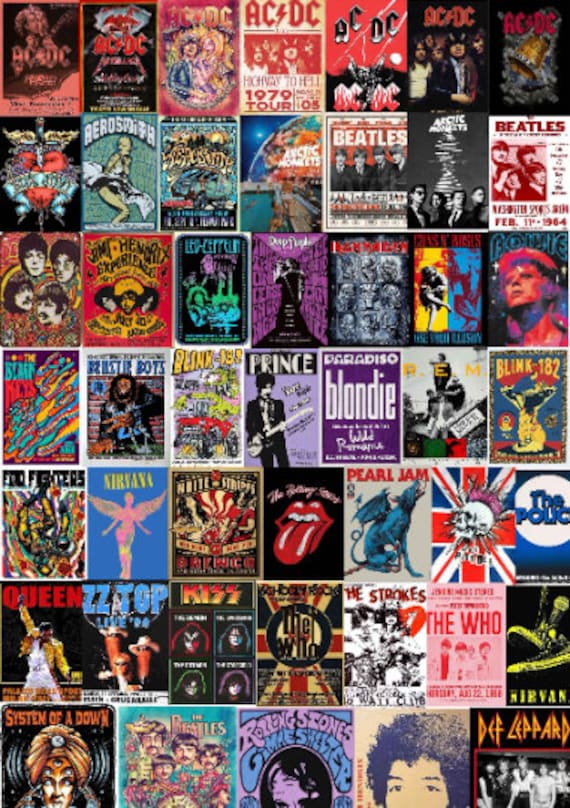This vertically-oriented image is a vibrant, borderless collage consisting of 49 covers, arranged in a 7x7 grid. Each cover represents album art or promotional material for various iconic rock and roll bands and artists. The first row features exclusively AC/DC covers, predominantly in red and black tones. The second row includes Aerosmith and several Beatles covers. Moving down, notable artists such as Jimi Hendrix, Led Zeppelin, David Bowie, Beastie Boys, Blink-182, Prince, and Blondie are displayed. Further rows showcase bands like Foo Fighters, Nirvana, Kiss, Pearl Jam, The Police, Queen, ZZ Top, The Strokes, The Who, System of a Down, Rolling Stones, and Def Leppard. The collection features a blend of color illustrations and color photography, offering a visually rich homage to rock and roll legends across the decades.